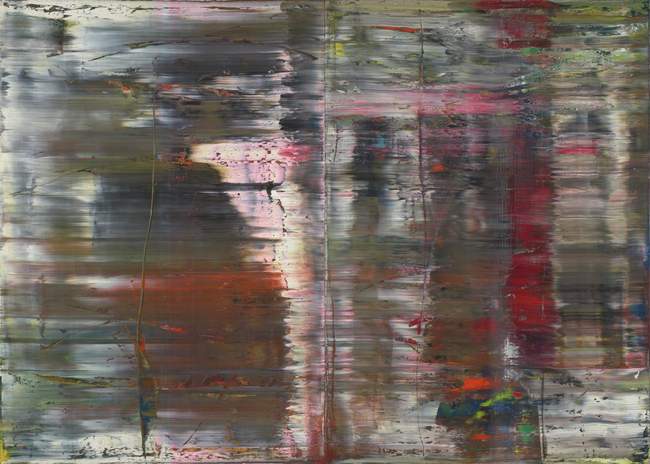The abstract painting is a captivating rectangular piece, likely executed on canvas or paper, with dimensions where the top and bottom are twice as long as the sides. Characterized by vigorous, random brush strokes made with large, strong sweeps, the artwork predominantly employs oil paints, creating textural ridges as the paint dried. The dominant strokes appear as chaotic lines, particularly featuring back-and-forth motions, forming two distinct columns of black paint, layered successively with splashes of red, black again, and green. Additional vibrant hues like orange, bright red, and lime green, along with streaks of pale off-white, offer a rich visual tapestry. Notably, the bottom right corner reveals dappled splashes of yellow, exposing the underlying canvas. While some colors merge and resemble a 'muddy' shade, there are clear, bright elements that seem to evoke a marshland scene, with reflections that mimic water surfaces. The detailed and layered nature of this painting invites prolonged contemplation, offering a striking and colorful visual experience.